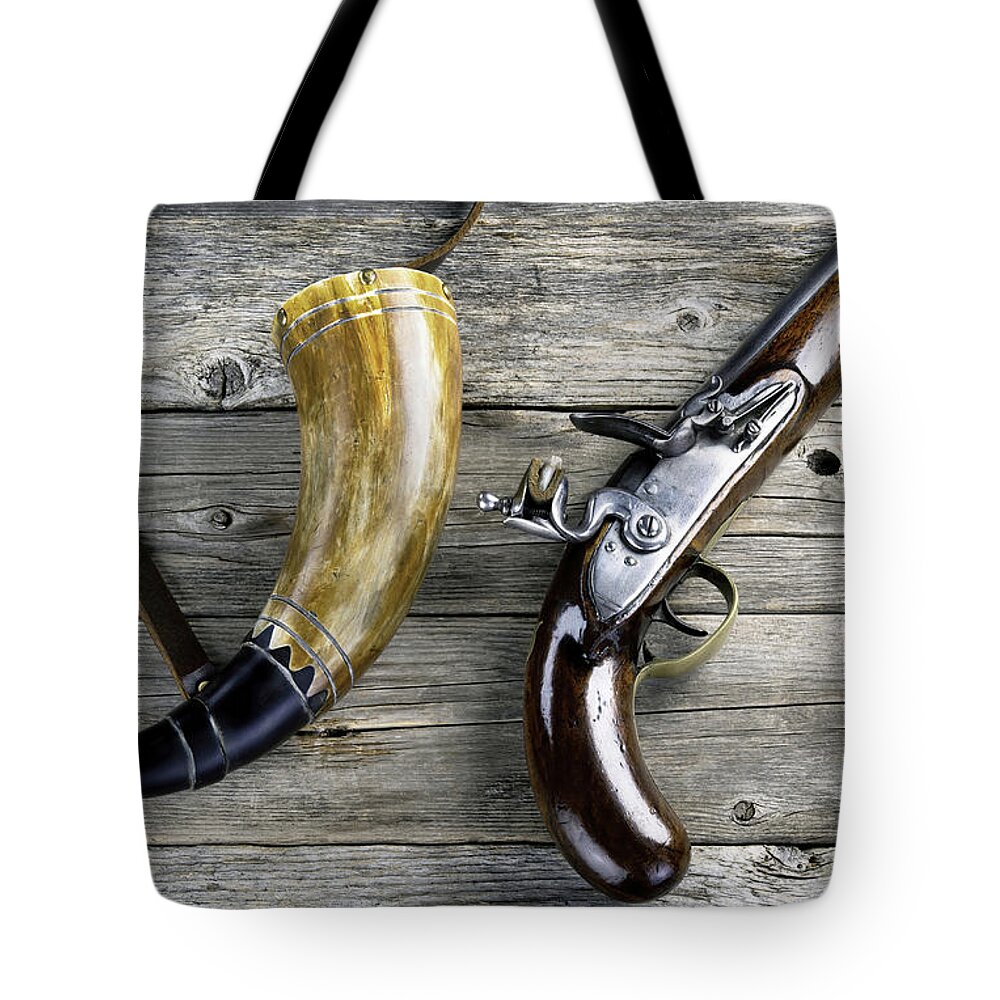This detailed close-up photograph showcases a beautifully preserved vintage gun and a bone-carved horn, both nestled on a rustic, dry gray wood planked table, reminiscent of a weathered picnic table. The image is printed on a tote bag with skinny black handles. The gun, likely from the 17th or 16th century, features a wooden body with silver hardware, and an eggplant-shaped barrel, suggesting a long rifle rather than a handgun. The gun is extremely shiny and in excellent condition, with distinguishing clips and possibly a brass piece that can be pulled back to shoot. Accompanying the gun is a well-polished bone horn, adorned with a black mouthpiece and a leather carrying strap. The horn is tan with a shiny, well-maintained surface. Both items exude a sense of Western historical charm, impeccably captured against the rustic backdrop.